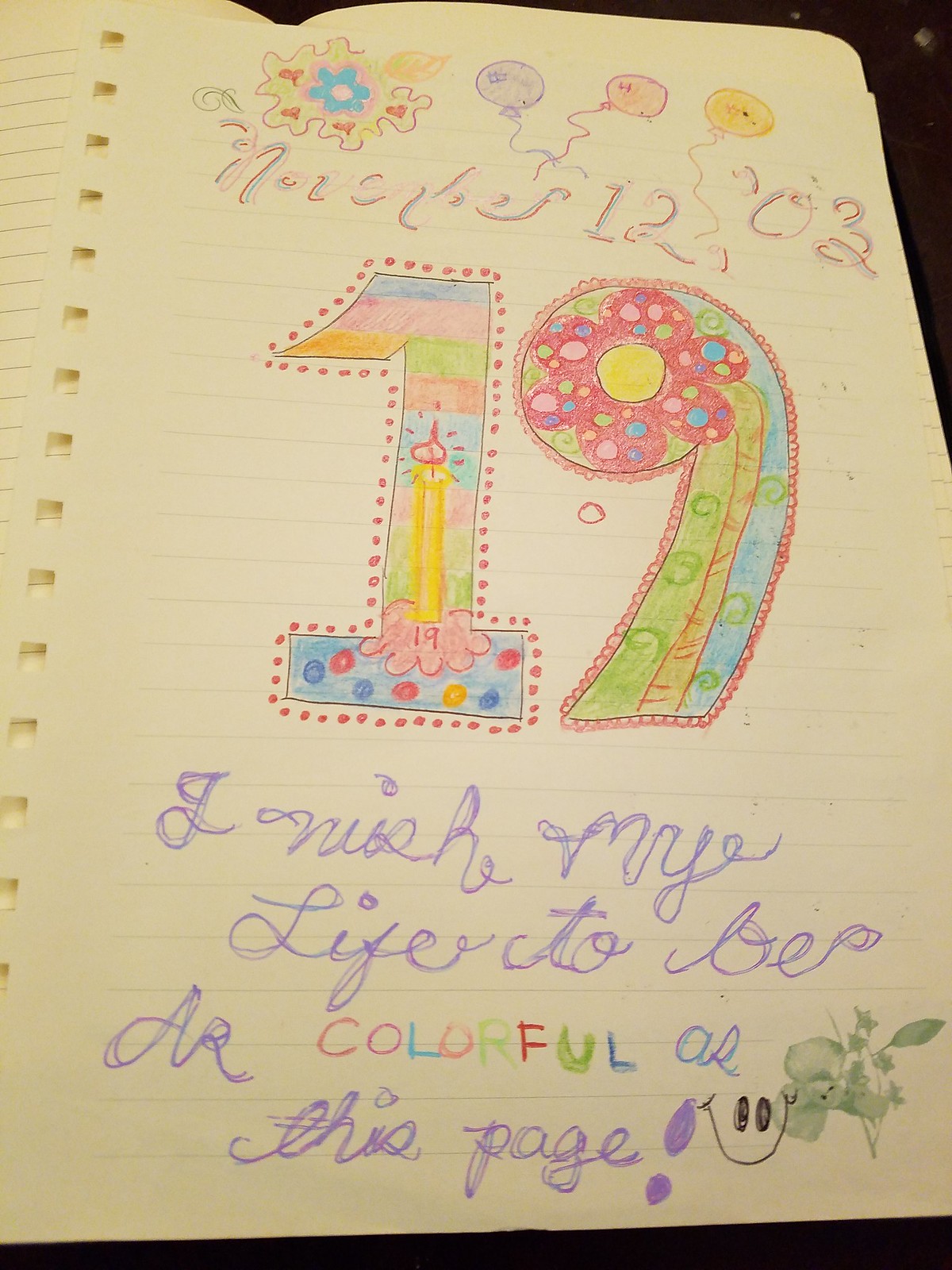This image showcases a hand-decorated journal entry on a light yellow, lined, vertically-rectangular spiral-bound page. At the very top, there is a flower with yellow petals, a blue center, and red hearts on the petals, next to three side-by-side balloons colored purple, pink, and yellow. Below, the date is written in script as November 12, '03. 

Prominently in the center of the page, the number "19" is drawn in large, vibrant digits. The "1" is adorned with a candle inside, surrounded by dots, with a small flower that has "19" written inside. The "9" contains a pink six-petal flower with a yellow center and has red lace-like accents around it. Surrounding the decorations inside the "1" and "9" are various colored stripes and additional floral elements. 

At the bottom of the page, written in colorful lettering with each letter in a different color, is the message, "I wish my life to be as colorful as this page," accompanied by a simple smiley face. The artwork seems to be created with colored pencils or crayon, adding a vivid and cheerful touch to the journal entry.